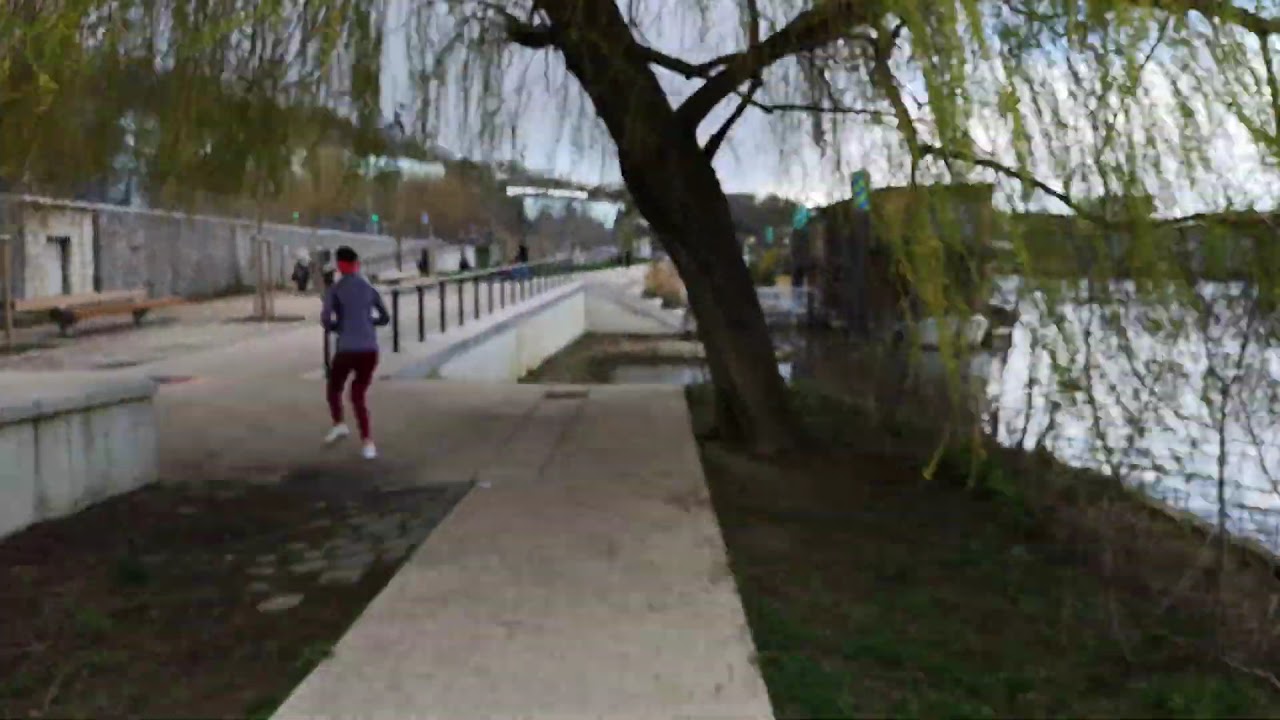This image depicts a detailed scene captured in a color landscape photograph, focusing on a riverbank pathway. The main feature is a light gray concrete walkway veering slightly to the left, running alongside a river on the right, bordered by a low guard rail. A jogger is centered to the left, dressed in red pants, a blue long-sleeve shirt, white shoes, and a red headband, viewed from behind. A large weeping willow tree with hanging green branches dominates the mid-ground, its foliage partially obscuring a small shack underneath. The background features a gently rising hill to the far left, peppered with indistinct buildings against a partially cloudy sky. Concrete structures, including a retaining wall and a sitting area, line the path on the left. The scene is framed in a photographic style of representational realism, capturing the serene riverside ambiance.